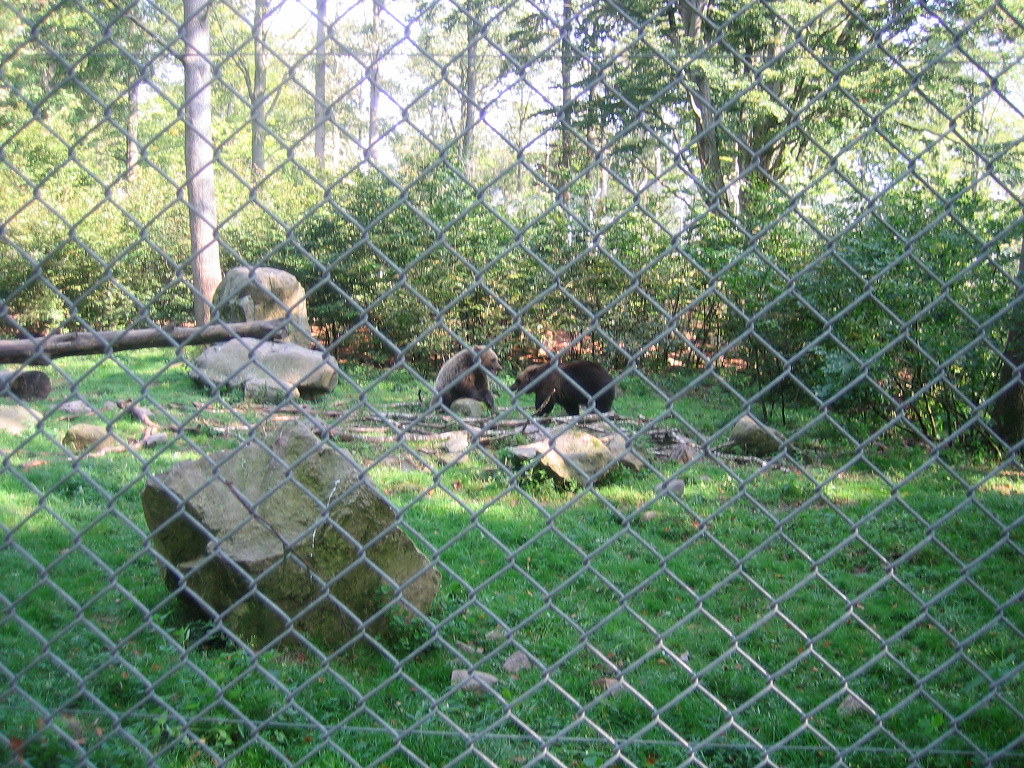An outdoor zoo enclosure is visible through a chain-link fence that covers the entire image. Inside this enclosure, two brown bear cubs appear to be playfully interacting, facing each other but not touching. They are surrounded by large boulders, including a prominent one in the foreground near the fence and several scattered throughout the area. A large log lies across one of these rocks to the left of the bears. The enclosure features lush green grass, along with numerous trees and bushes that contribute to a well-shaded environment. Some tree branches and broken limbs are also visible on the ground, adding to the naturalistic setting. Sunlight filters through the leaves, indicating it's daytime, and the overall scene provides a glimpse into the bears' habitat, highlighting the blend of rocks, vegetation, and playful wildlife.